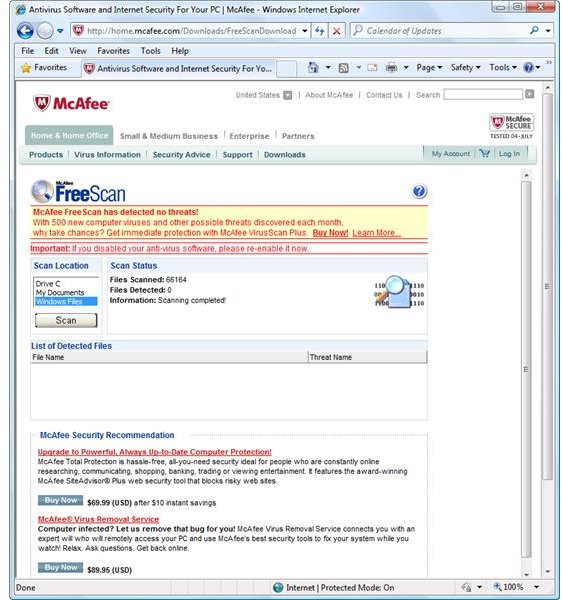In this screenshot, we see a webpage set against a predominantly white background with a blue heading at the top. In the upper left corner, there is an Internet Explorer icon. To the right, in black text, it reads "Antivirus Software and Internet Security for Your PC - McAfee Windows Internet Explorer." Below this heading, there is a white address bar displaying “http://home.mcafee.com”.

On the main portion of the screen against the white background is the McAfee icon, which resembles a red shield, and to its right, there are red block letters spelling out "McAfee". Below these, there is a menu bar featuring categories labeled "Home and Home Office", "Small and Medium Business", and "Enterprise and Partners".

Further down, in large blue text, it reads "McAfee Free Scan". Beneath this, in red text against a yellow background, is a message stating, "McAfee Free Scan has detected no threats". Below this message, a line of text reads, "With 500 new computer viruses and other possible threats discovered each month, why take chances?"